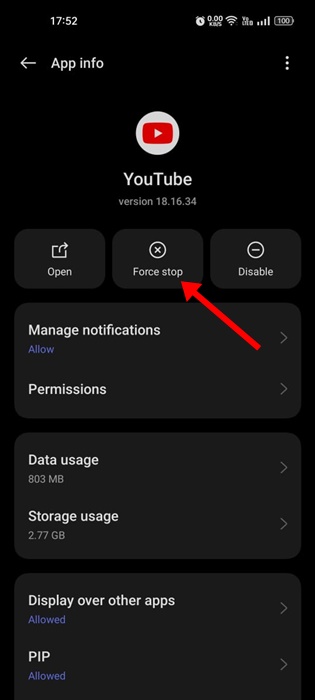The screenshot showcases the "App Info" page for the YouTube application on a smartphone. The page is set against a black background with "App Info" written in white at the top, accompanied by a left-pointing arrow and three vertical dots on the right side for additional options. Immediately below, the recognizable YouTube logo—a red play button inside a white circle—is displayed alongside the app's name "YouTube" and its version number "1.8.16.34."

Underneath the logo and name are three actionable buttons: "Open," "Force Stop," and "Disable." Notably, a bright red arrow points to the "Force Stop" button, indicating that this screenshot aims to guide the user on how to force stop the YouTube application.

Further down, additional settings are listed, such as "Manage Notifications" with a status of "Allow," "Permissions," "Data Usage" showing "803 MB," "Storage Usage" indicating "2.77 GB," "Display Over Other Apps" with a status of "Allowed," and "Picture-in-Picture (PIP)" also marked as "Allowed." Each of these settings features a right-facing arrow, signifying that they are clickable for further configuration. This screenshot serves as a detailed guide to manage YouTube app settings, particularly focusing on force stopping the application.